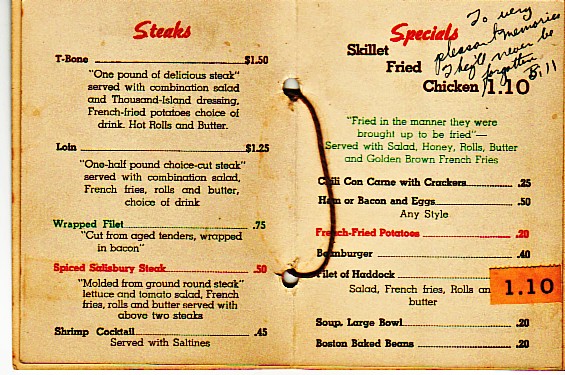This vintage menu, seemingly aged with time, displays a personal note in elegant handwriting on the upper right-hand corner that reads, "To very pleasant memories, they'll never be forgotten, Bill." The menu itself is accentuated with a light beige backdrop and two pages bound together by brown string threaded through two holes. It features a blue border that subtly frames the text.

### Page 1:
- Steaks:
  - T-bone: $1.50
  - Loin: $1.25
  - Wrapped Filet: $0.75
  - Spiced Salisbury Steak: $0.50
  
- Shrimp Cocktail: $0.45

### Page 2:
- **Specials** (marked in red):
  - **Chicken Fried Chicken** (in black letters): $1.10
  - In green letters, a whimsical description reads, "fried in the manner they were brought up to be fried, served with salad, honey, rolls, butter, and golden brown french fries."

  - In black letters:
    - Chili Con Carne with Crackers: $0.25
    - Ham or Bacon and Eggs, any style: $0.50

  - In red writing:
    - French Fried Potatoes: $0.20
    - A partially obscured burger priced at $0.40

  - Filet of Haddock with Salad, French Fries, Rolls, and Butter: $1.10 (in black letters with an orange tag)

  - Soup (Large Bowl): $0.20
  - Boston Baked Beans: $0.20